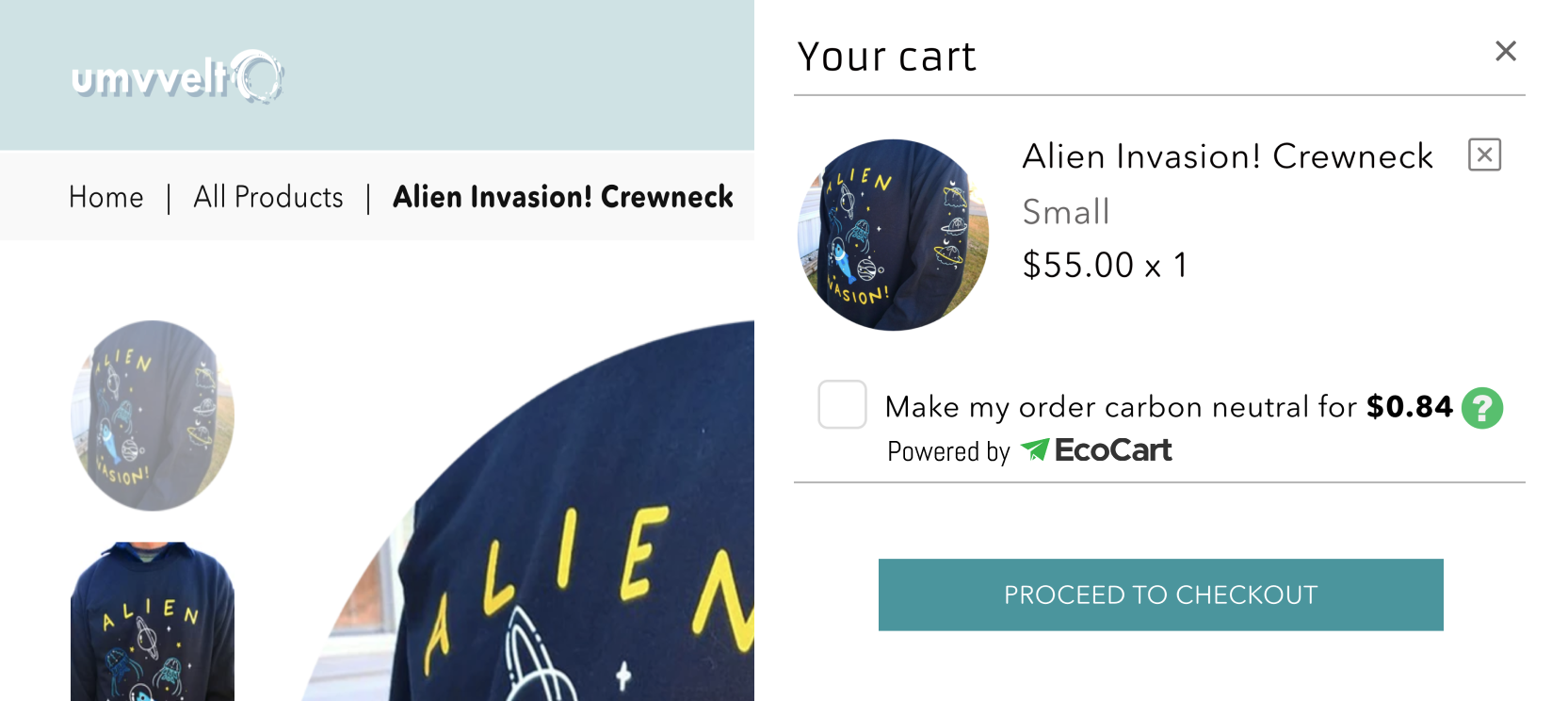A screen capture shows a mobile phone displaying a shopping cart on the Umvelt website. The shopper has selected an "Alien Invasion" crew neck sweatshirt in size small. The sweatshirt features the phrase "Alien Invasion" on the back, along with a cartoon depiction of a planet with rings and other celestial elements. The item in the cart is priced at $55. An option to make the order carbon neutral for an additional 84 cents is available. The screen also includes a prominent green button labeled "Proceed to Checkout."